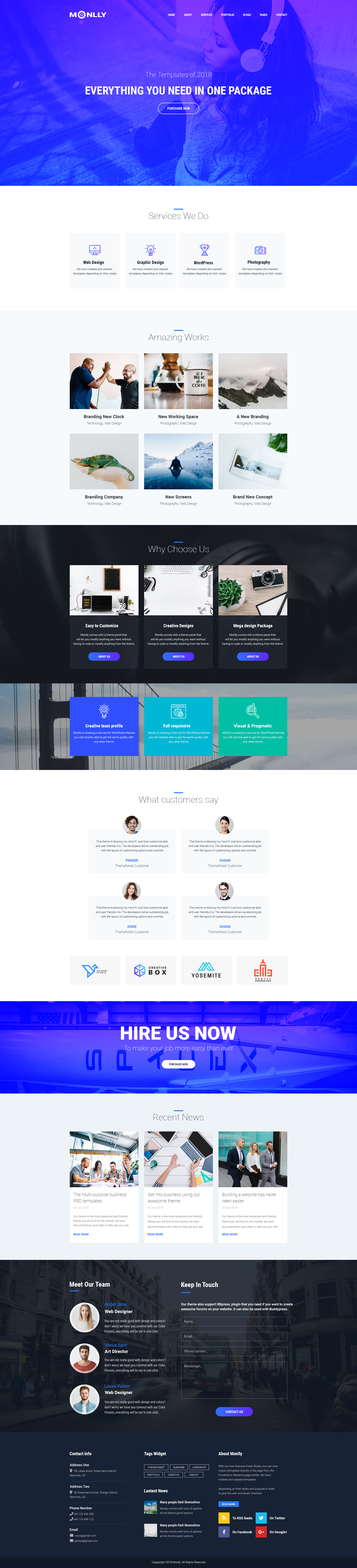This image displays an array of screenshots from a web design platform called Monly (spelled M-O-N-L-L-Y). The primary screenshot at the top showcases the main page of the website, which prominently features 2018 templates and a "Purchase Now" button, promising comprehensive solutions in one package. Beneath this, the site is segmented into various categories explaining the extensive services offered, showcasing impressive portfolio pieces, and highlighting customer testimonials that vouch for the company's excellence. Another screenshot delves deeper, presenting an option to hire Monly's services with a tagline emphasizing ease and efficiency. Further down, information is provided about the dedicated team behind Monly, along with multiple contact methods for inquiries and additional details.